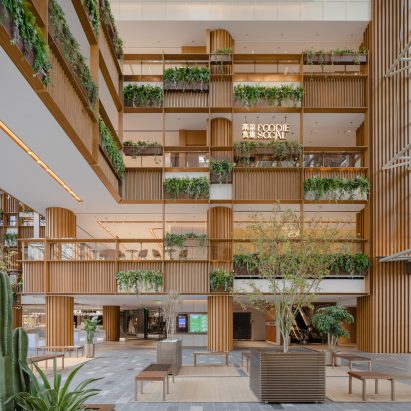This detailed image captures the sophisticated and modern interior of a high-ceilinged, four-story building, possibly a mall, hotel, or business center. The open-concept space features prominent light-colored wood paneling throughout, contrasted by white ceiling accents and light-colored carpeting on the ground floor. At the center of the image, a large wooden square planter showcases a robust tree, around which several wooden benches are placed, inviting visitors to sit and relax; a garbage can is also nearby. To the left in the foreground, a cactus and other green shrubbery accentuate the organic aesthetics. Each of the balconies on the levels above is adorned with various hanging plants and fern-like greenery, enhancing the fresh, natural ambiance.

On the third floor, an illuminated sign reading "Foodie SoCal" is displayed, complemented by Asian characters on its left, suggestive of a culturally diverse commercial environment. The design of the space is reminiscent of hotels like Embassy Suites, where room entrances open onto balconies overlooking the central atrium. Overall, the space exudes an air of modern sophistication and elegance, with abundant greenery that breathes life into the architecture.